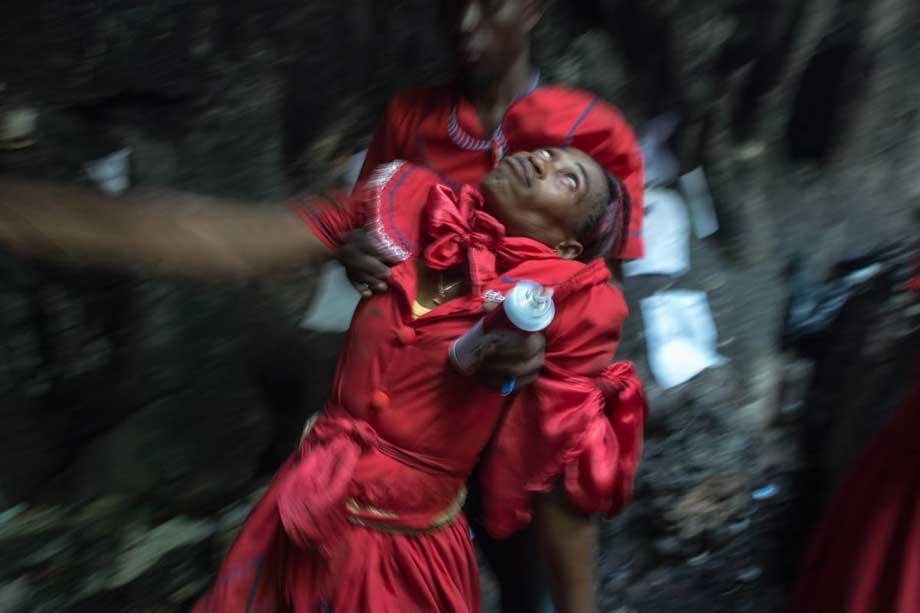The blurry, AI-generated or heavily filtered image depicts two individuals at the center, both dressed in elaborate, antique-style red attire. The foreground features a person in a flouncy red dress adorned with large buttons down the front, puffy sleeves with bows, and a v-neckline with a red bow at the collar. The dress, swaying slightly, creates pleats and folds, adding to the motion blur effect. This individual has dark skin and appears to be incapacitated or unsteady, possibly under the influence of a substance. Behind them, another figure, also in red, supports the person in the dress by holding them under their shoulders, suggesting an attempt to prevent them from falling. This second individual, whose features are less clear due to the blur, holds a can that looks like spray paint or an aerosol in their left hand. Both individuals seem to be in a dark, indistinct environment with hints of gray, burgundy, and black tones, which might evoke the sense of them being in a ditch or an unknown, shadowy location.